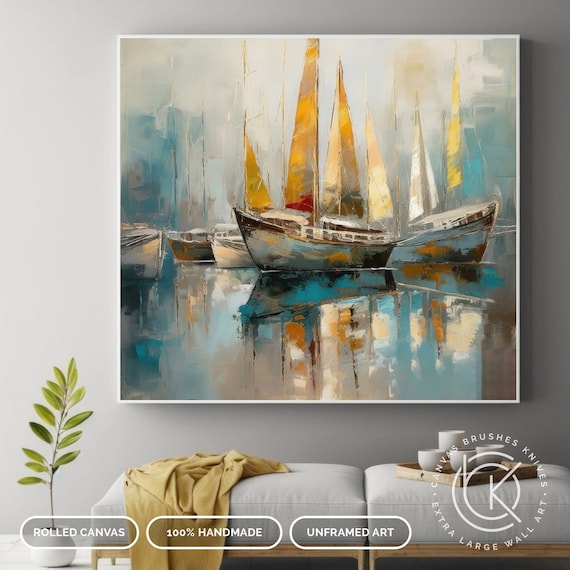The photograph captures a serene and detailed interior scene featuring a grayish wall with noticeable shading differences; the left side is brighter while the right side fades into a shadow. Mounted on this wall is a striking painting of a harbor filled with approximately five sailboats, depicted with abstract, blocky forms. The painting, framed by a thin, white border, showcases ships with gold-colored sails reflected in a deep blue and turquoise sea under a sky with patches of white. Below the painting, two small, backless stools with gray cushions are arranged, one adorned with a tan jacket or blanket and the other holding a tray with coffee cups. To the left beneath the painting, a round white planter holds a single green frond with little leaves. At the bottom of the painting, text reads "rolled canvas, 100% handmade, unframed art," accompanied by an oval logo on the right incorporating the letters R and K, encircled by phrases such as "canvas, brushes, knives, extra large wall art."